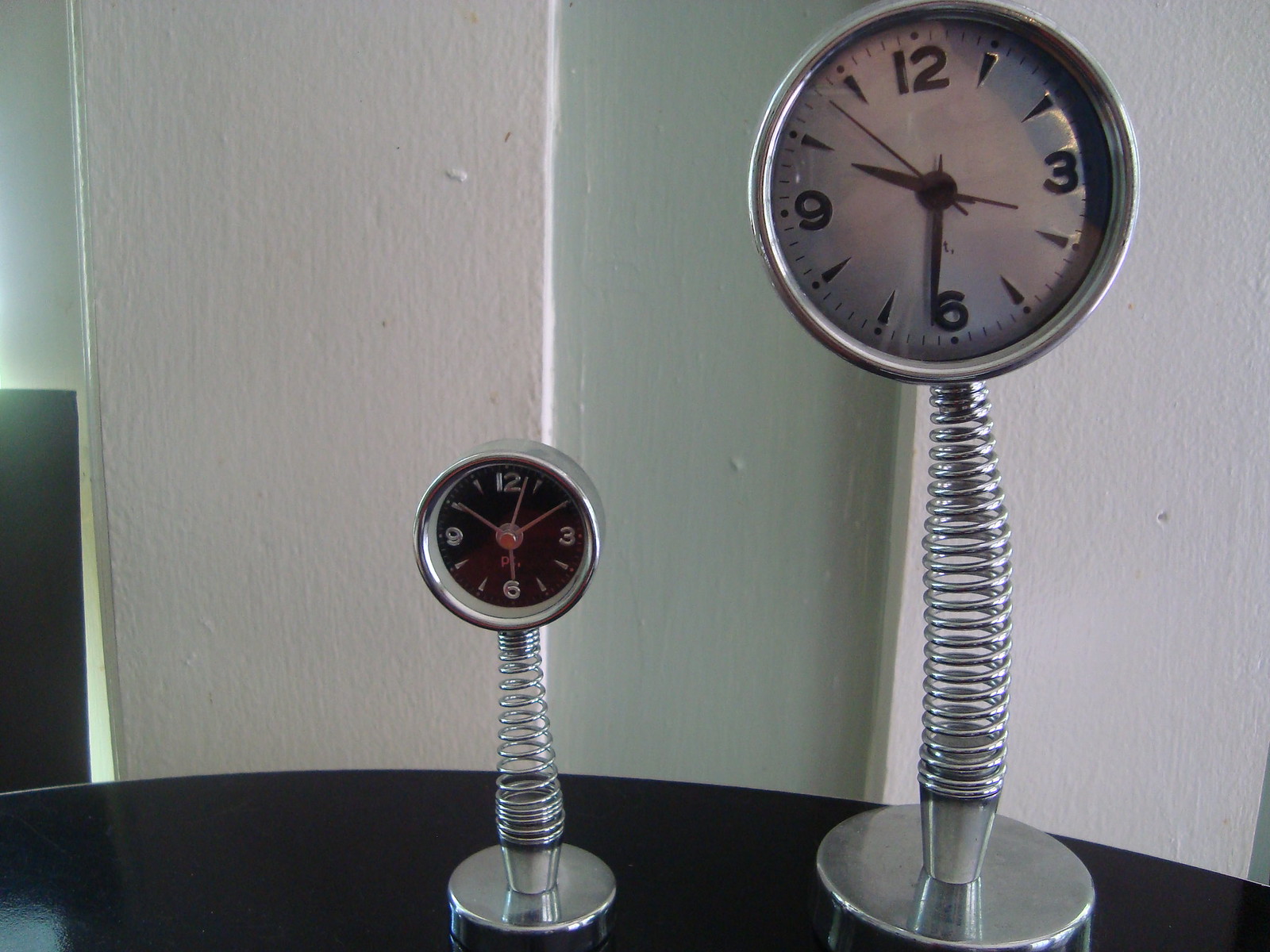This image features two clocks displayed on stands that resemble flexible springs. Both clocks are set atop a black table. The background comprises a white section that appears to be part of a doorway.

The smaller clock, standing approximately four to five inches tall, has a dial comparable in size to a small saucer. The clock is predominantly silver, with a striking black face. It displays the time as around 6:03. This clock has four hands, including the second hand, while the purpose of the additional hands remains unspecified.

In contrast, the clock on the left is significantly taller, standing at about 10 inches or more. Its clock face, roughly the size of a small dinner plate, is white and shows the time as 10:31. Similar to the smaller clock, it also features four hands. The dial retains a minimalist design, with only the numbers 12, 3, 6, and 9 marked, and lines serving as placeholders for the other hours. The numbers are in black, enhancing the contrast against the white face.